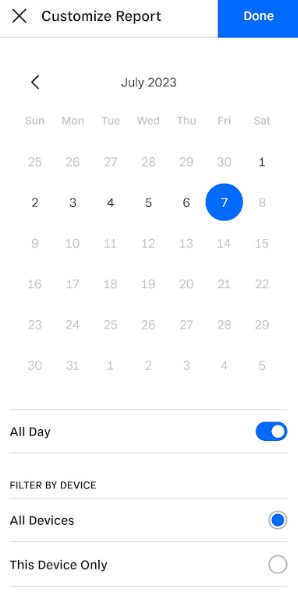The image is a screenshot from an application in portrait orientation, featuring a clean and minimalistic interface. At the top of the screen, the title "Customize Report" is displayed in bold black letters. On the left side of the title is a black 'X' icon, likely intended to clear or close the window. On the right side, there is a cobalt blue rectangular button with the word "Done" in white text.

Directly below the header is a thin gray line that separates the rest of the screen. The main content is a calendar displaying the entire month of July 2023, with days of the week listed from Sunday to Saturday. Next to the month name "July" is a back arrow, suggesting the ability to scroll to different months. Within this calendar, Friday the 7th is distinctly highlighted with a solid cobalt blue circle.

Beneath the calendar, another thin gray line divides the screen into several rows. The top row is labeled "All Day" and includes a toggle button, which is toggled on, represented by a white circle on a cobalt blue oval background. Below this is the "Filter by Device" section, which provides two radio button options: "All Devices" and "This Device Only." The "All Devices" radio button is selected, indicated by a solid blue circle in its center, while the "This Device Only" option is unselected, marked by a gray outline circle. 

This detailed interface layout helps users customize their reports effectively within the app.